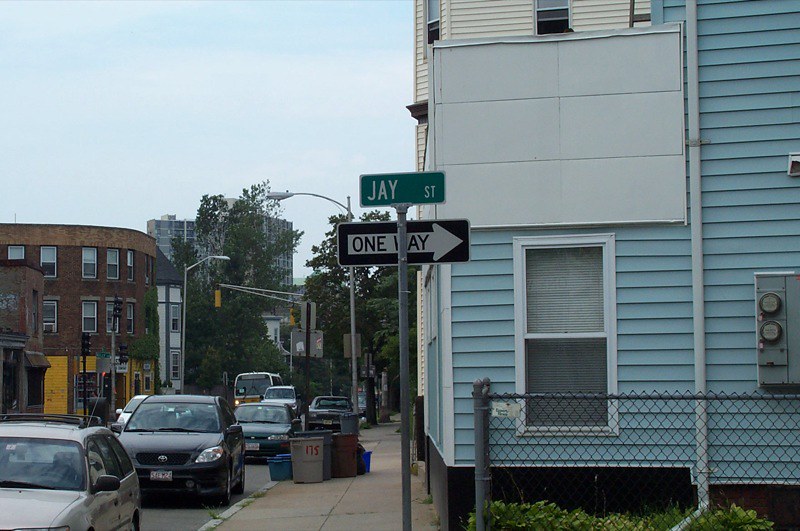This color photograph captures a bustling urban scene, possibly within a small neighborhood or city. In the top left corner, a rectangular section reveals a clear blue sky, contrasting against the built environment. Dominating the right side of the image, a prominent blue building is partially visible, with segments obscured by a chain-link fence. Above the fence, electric meters are discernible, adding to the urban aesthetic.

Adjacent to the meters, a window peeks through, framed by white paneling that provides a stark contrast to the blue facade. The lower portion of the building is crisscrossed by the chain-link fence, which adds texture to the foreground.

Near the center of the image, street signs stand in front of the blue building, indicating the location as J Street. The street sign also signals a one-way street pointing to the right. In the lower left and extending into the background, another multi-story building is partly visible, likely around three stories high. The street in front of this secondary building hosts several parked cars, all oriented towards the camera, contributing to the lively, urban atmosphere.